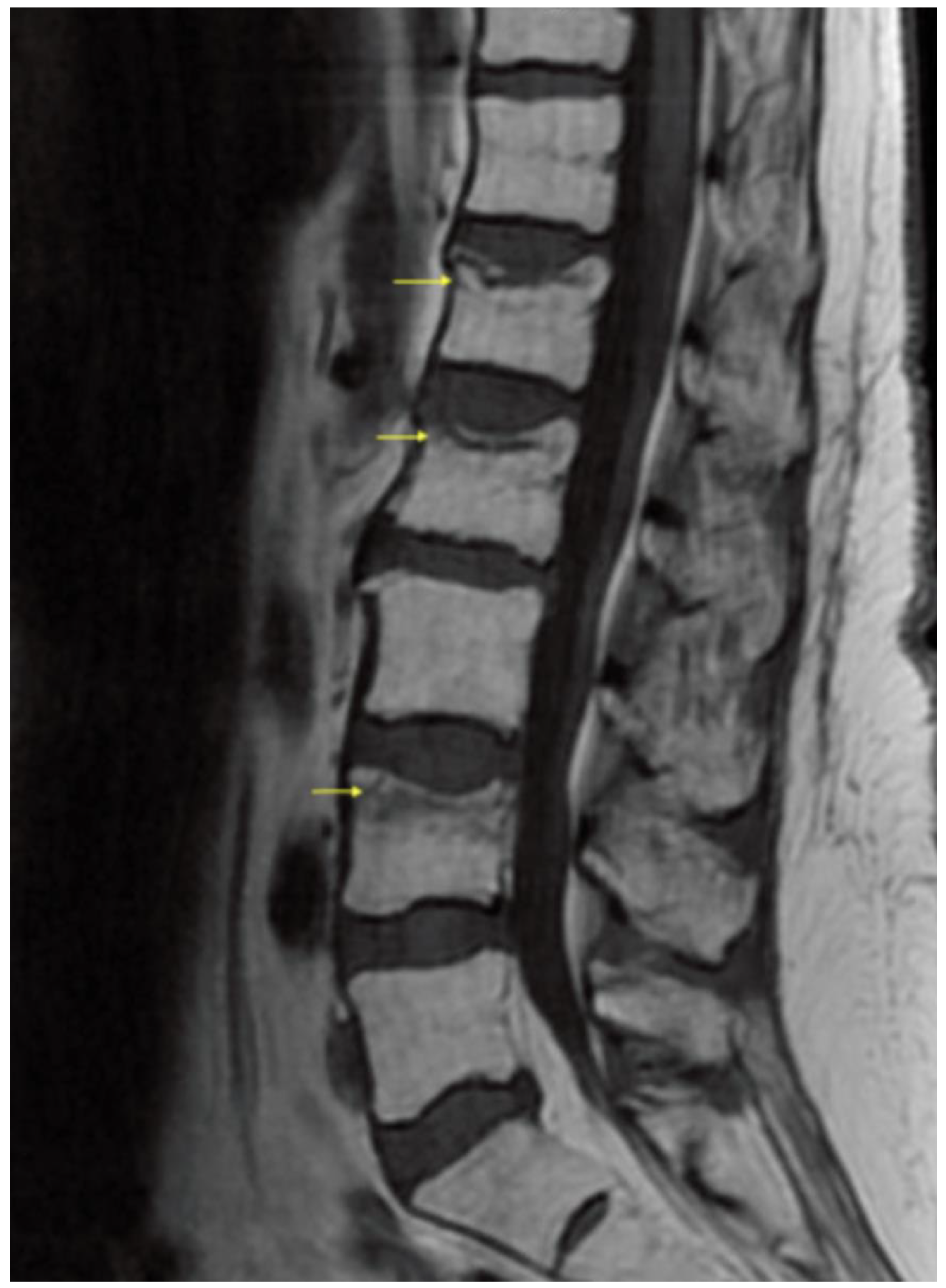This image is a detailed x-ray of a spine in a black and white (or black and grayish white) color scheme. The primary focus is on the spine, which appears healthy and straight, with clear visibility of the spinal cord and adjacent structures. The vertebrae run down the center of the image and have a curved alignment, showing a series of discs that provide cushioning between each vertebra. Alongside the spine, there are repetitive gray and black oval shapes, resembling a tire tread pattern. Notably, there are small yellow arrows pointing to three specific vertebrae - two at the top and one midway down. These arrows highlight areas with possible issues, such as fractures or other anomalies, as indicated by the darker shading on these vertebrae. The image also features a white area extending diagonally from the upper right to the lower right, contrasting with the predominantly dark left side. Overall, the x-ray depicts a well-maintained spinal structure, with minor indentations but no signs of severe conditions like scoliosis or herniated discs.